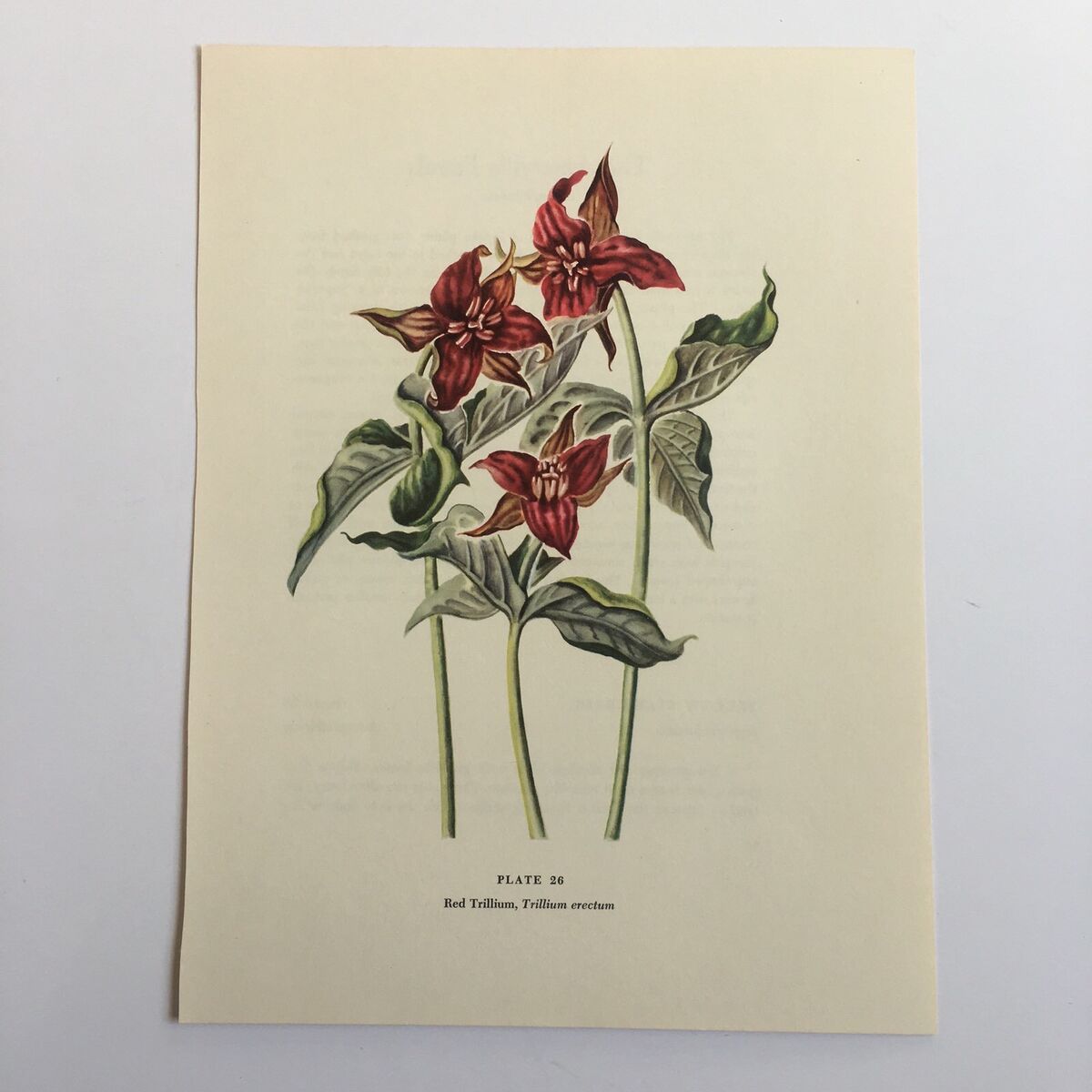The image features a detailed illustration of three red Trillium (Trillium Erectum) flowers, labeled as "Plate 26." Each flower is characterized by five petals with a seeded center and is supported by a long green stem with three somewhat curled green leaves. The illustration is presented on a slightly yellowed, vintage-looking piece of paper that is translucent enough to reveal faint, unreadable text beneath it. Despite the simple nature of the composition, with the flowers on a white card situated against a white background, the intricate details of the flowers and the vintage quality of the paper provide a sense of elegance and botanical accuracy.